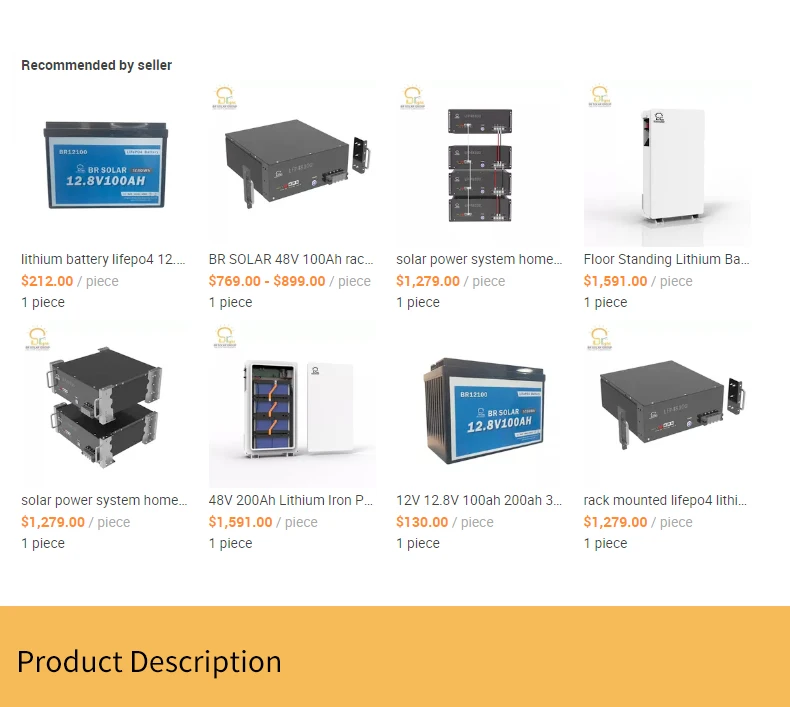A screenshot of an e-commerce website displaying a selection of recommended products for sale. At the top left corner, a heading reads "Recommended by Seller." Beneath this heading, there are two rows of products arranged in a four-column grid, making up a total of eight items. The products and background elements are set against a simple white backdrop, drawing attention to the items themselves.

In the first row, the products appear to be energy-related. The first item is labeled "Lithium Battery Life PO412..." and is priced at $212 per piece. The accompanying image shows a black battery with a white and blue label. The second item is titled "BR Solar 48 Volt 100 Amp RAC..." and is priced between $769 and $899 per piece. Its corresponding image depicts a black rectangular device. Each product in both rows follows a consistent format, displaying an image at the top, followed by a title, price, and quantity information.

At the bottom of the screenshot, there is an orange box with the text "Product Description" written in black letters on the left side. The website appears minimalistic and functional, focused entirely on showcasing the products without additional distractions or elaborate design elements.